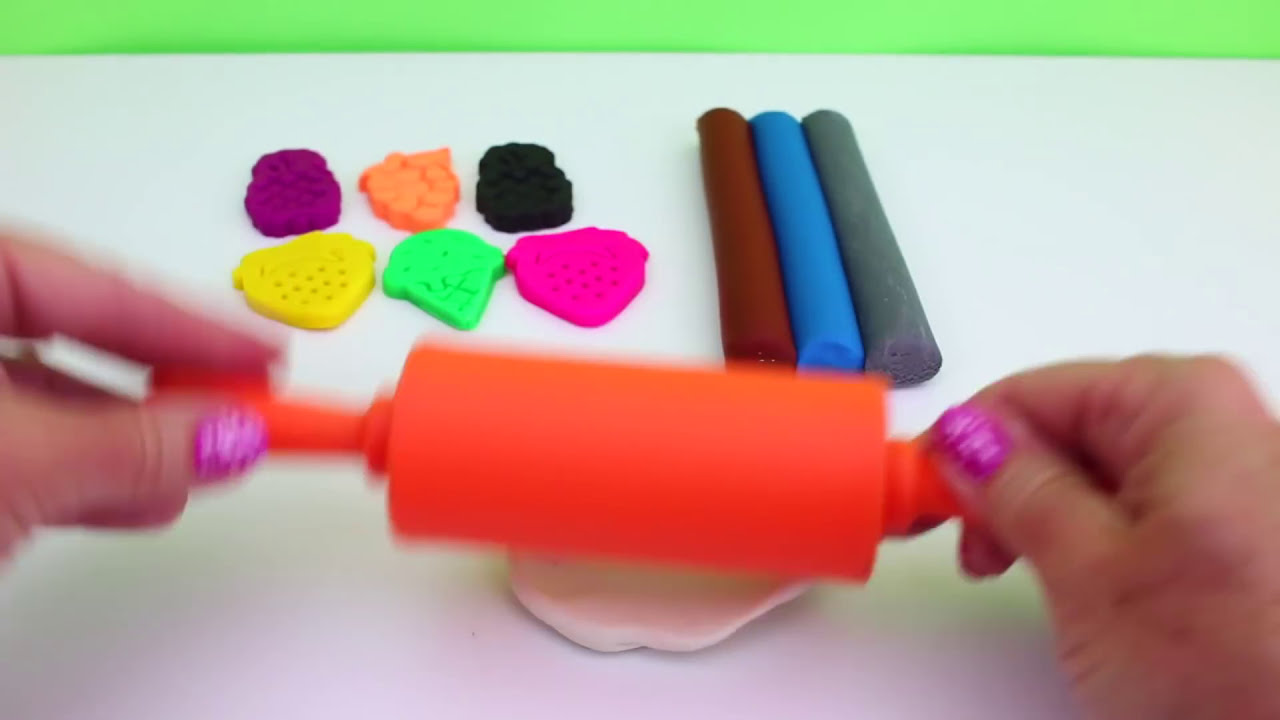The photograph depicts a pair of hands with purple, shimmering nail polish, holding a small, orange rolling pin, which is being used to roll out white clay. The focus of the image is on various clay items positioned in the background, while the hands and roller appear blurry. Behind the rolling pin, three cylindrical clay strips in brown, blue, and gray are visible. To the left, there are six molded clay objects, arranged with three on the top and three on the bottom in colors like purple, orange, black, yellow, green, and pink, resembling berries or other shapes. The scene is set against a white surface with a lime green border at the top.